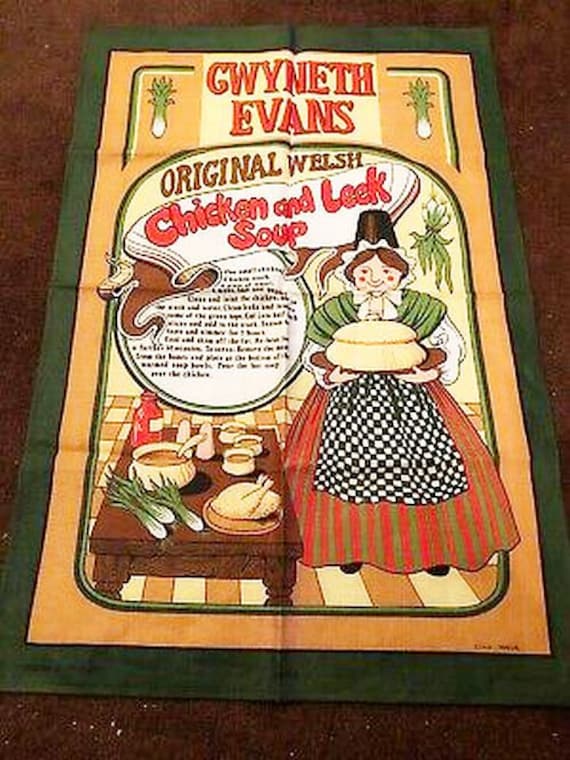The image displays a vertically oriented rectangular tapestry set against a weathered red, wooden background. The tapestry, defined by a green border and a central yellowish-orange rectangle, features a detailed design. At the top, within a white box adorned with red lettering, it reads "GWYNETH EVANS." Below, framed text announces "ORIGINAL WELSH CHICKEN AND LEEK SOUP." Occupying the lower right section is an animated depiction of a woman dressed in prairie-style attire, including a checkerboard apron, shawl, and a tall pilgrim-like hat, holding a large yellow cake on a brown dish. To her left, a table displays a spread that includes a plate with a chicken, stalks of leeks, and a pot of soup. The tapestry also includes unreadable instructions for soup preparation, adding a touch of authenticity to its promotional design.